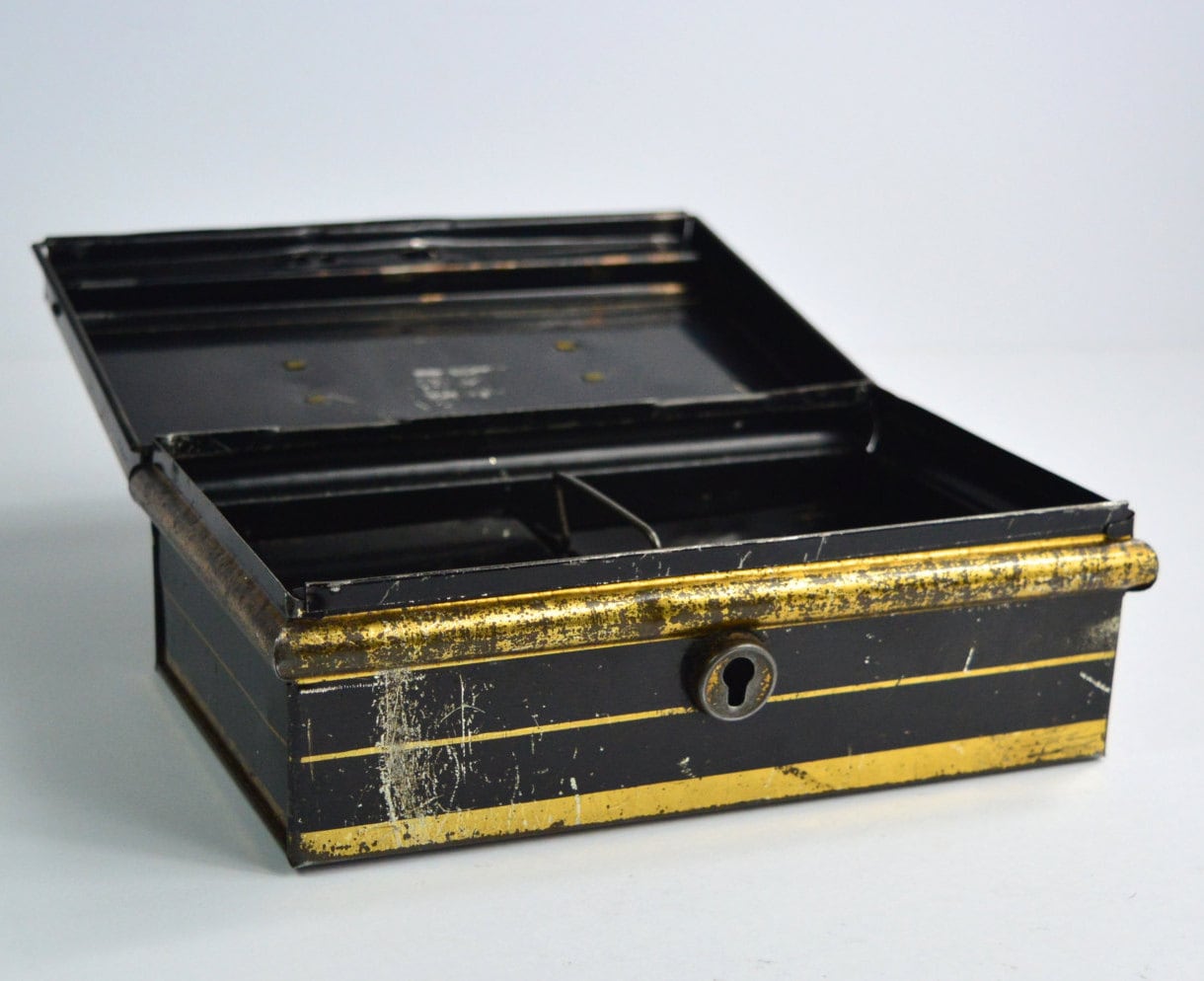This image features an antique metal money box set against a solid light gray background. The box is rectangular and primarily black, with significant wear and scratches revealing the metal beneath. It is adorned with gold embellishments, including a gold border around the top, sides, and bottom, though much of the gold paint is faded or scratched away, exposing the worn black surface underneath. The lid, held by a hinge, is open, displaying two compartments divided by a central bar. The interior appears black with some blurry white writing on the underside of the lid and four visible screws. A vintage style keyhole is positioned on the front, though no key is present. The box’s aged appearance, with its scratched and faded paint, hints at its historical value and antique charm.